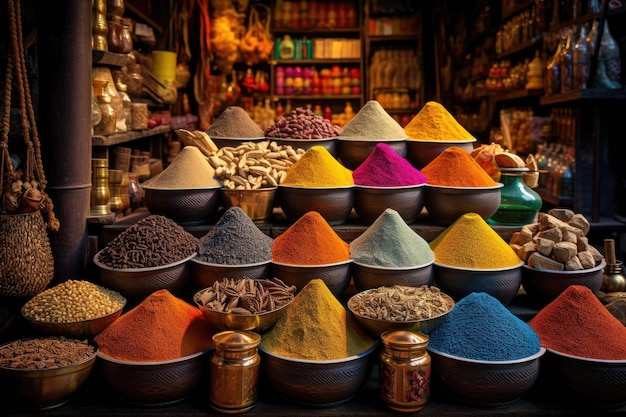The image features a vibrant market stall, likely that of a spice or dye shop, filled with an array of colorful and varied items. At the forefront of the stall, a tiered table displays large black ceramic bowls on multiple levels, each containing different kinds of vibrant spices or dyes. Starting from the left, a silver bowl is brimming with dried round nuts or fruit. Behind it, another bowl is filled with round yellow balls. Adjacent to this, a bowl mounded with vivid orange powder sits next to another bowl containing more dried fruit. 

The background of the shop is lined with shelves, neatly arranged with various copper, bronze, and glass utensils and pots, along with an assortment of bottles and other objects. These shelves flank both sides of the center area and contribute to the rich, eclectic atmosphere of the market stall. Hanging in the left-hand corner is a beaded bag, adding a touch of artisanal charm to the scene. Central to the image are the bowls filled with multicolored substances, ranging from orange, pink, and yellow to blue, light green, gray, and brown. Some of these items are solid condiments or large spices and potentially other food items, underscoring the diverse and rich offerings of the market stall.